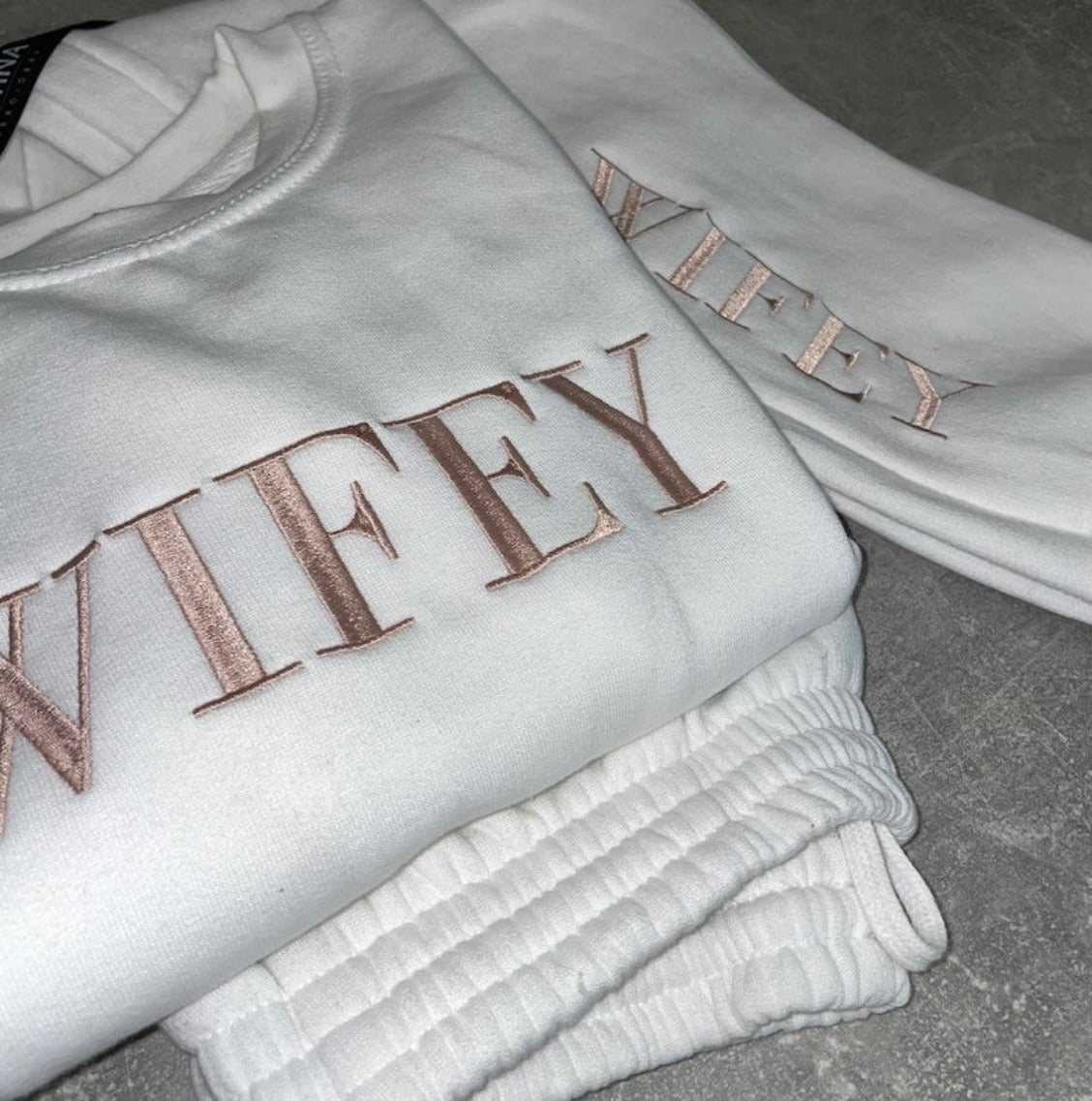The image features a stylish white sweatsuit comprising a sweatshirt and sweatpants, both meticulously folded and placed atop one another. The fabric is a pristine white or perhaps a creamy white shade, providing an elegant backdrop for the eye-catching champagne or rose gold-colored embroidery. The embroidery spells out "WIFEY" in large, glittery, serif-font block letters. On the sweatshirt, the word "WIFEY" is prominently displayed across the front, while it runs down the leg of the sweatpants. The ensemble is laid out against a solid gray surface, which could be a floor or a tabletop, adding a sleek contrast to the attire. The photo captures the outfit in a flash, cutting off part of the "W" on the sweatshirt and showing the fold of the pants with the waistband closest to the camera. The luxurious fabric and sophisticated design suggest it is more suited to a dressy casual setting rather than for gym activities.